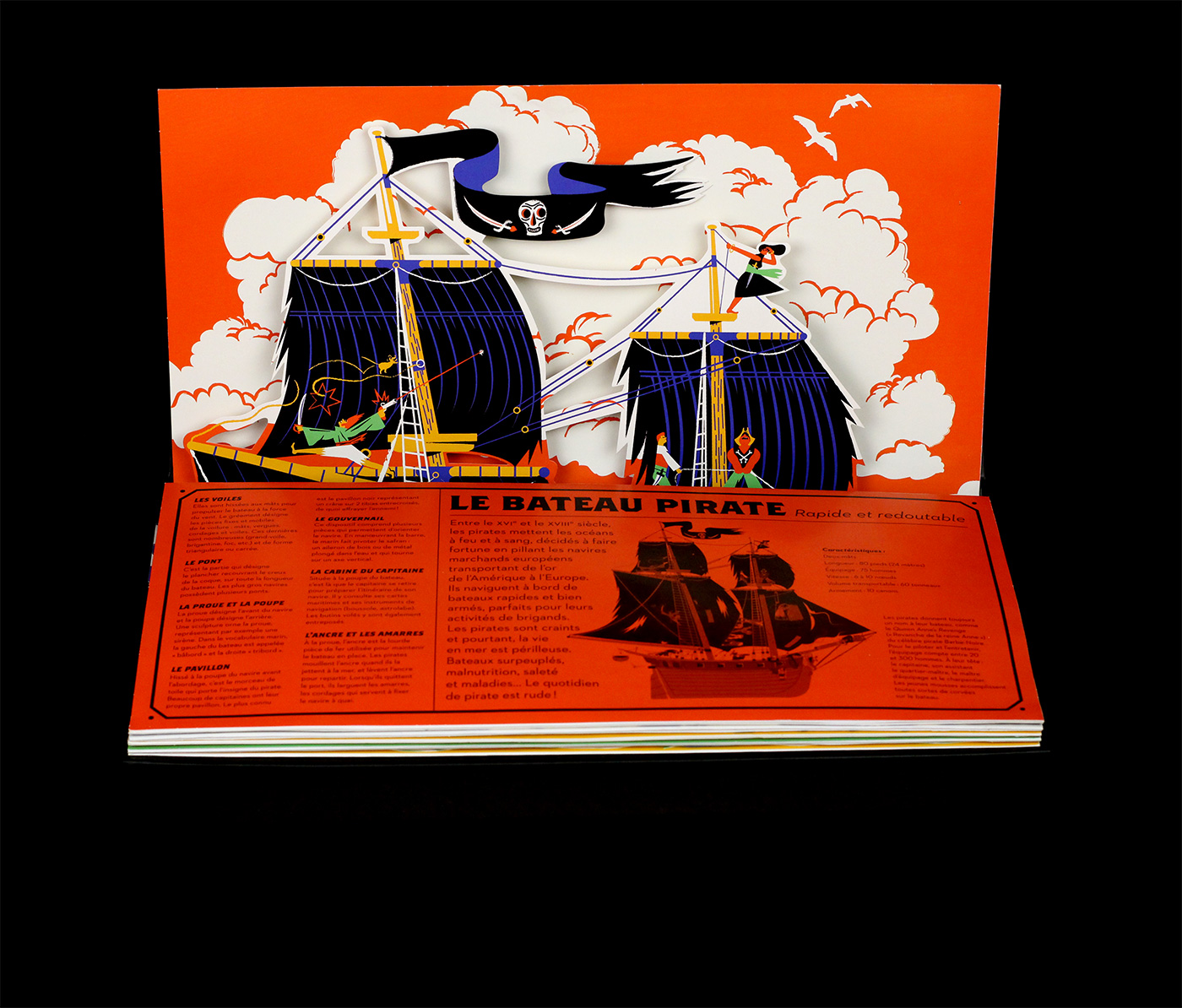The photograph depicts a vibrant pop-up book set against a black backdrop, featuring pages that unfold to reveal a detailed, cartoon-like scene of pirate adventures. The book is primarily orange in color and contains text in French, prominently featuring the title "Le Bateau Pirate." The upper portion of the open pages showcases a three-dimensional pop-up of two animated pirate ships with sails that are predominantly black with blue highlights. The masts are wooden-colored, and intricate white rigging is visible. One ship displays a waving pirate flag adorned with a skull and crossed swords. The backdrop includes an orange sky with scattered white clouds and silhouettes of white seagulls. On the main mast of the second pirate ship, a pirate figure stands, dressed in a skirt that blows in the wind with a distinct green sash around their waist. The opposing page exhibits an illustrated sketch of a pirate ship, along with additional French text, though the wording is too fine to discern. This richly detailed book page combines elements from all three captions to provide a cohesive and immersive description.